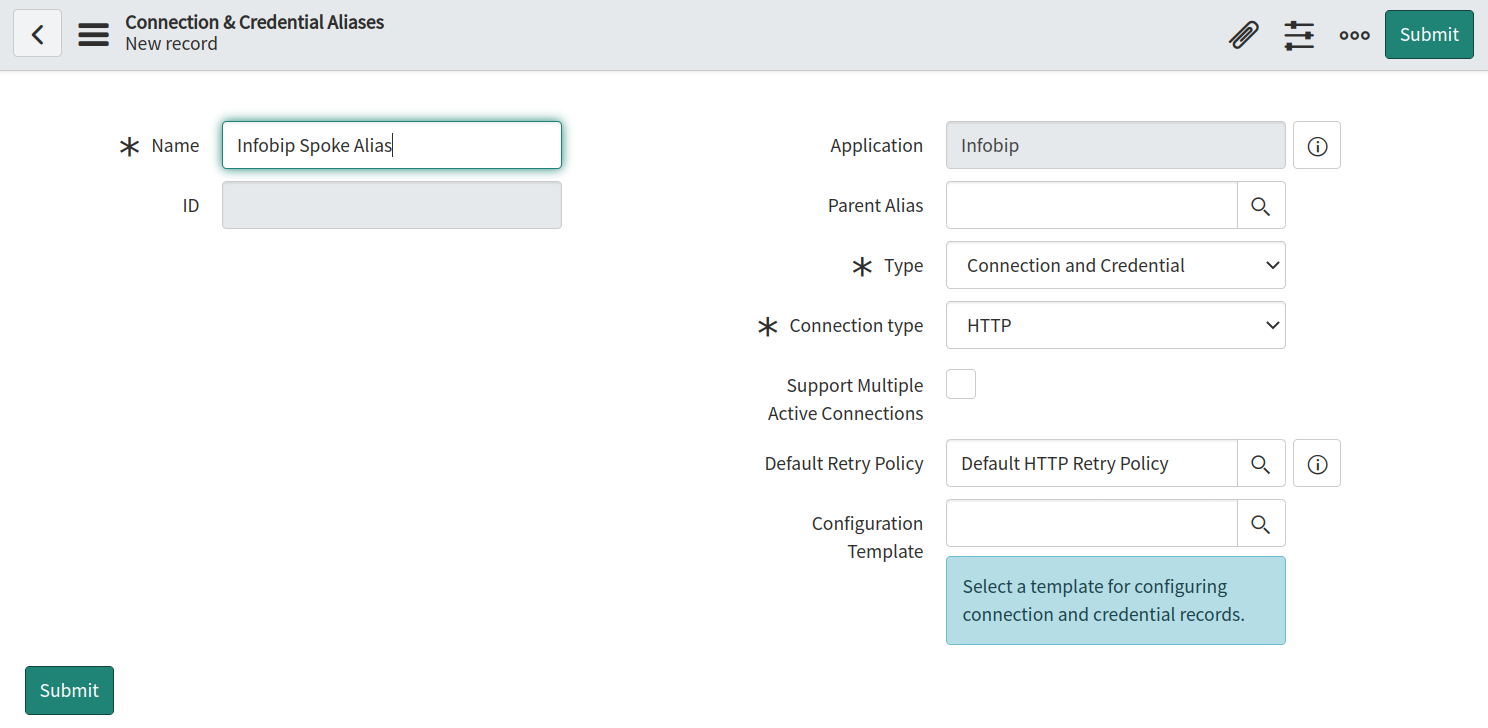The image displays a user interface composed of multiple distinct sections and elements:

- On the left-hand side, there is a lighter gray box marked with a black arrow.
- Adjacent to this, three bold, black horizontal lines are present.
- Beside these lines, the text reads "Connection and Credential" as aliases.
- Below this text, there is a label indicating "New Record."
- On the right side, an icon resembling a paper clip is visible.

Further to the right:
- There are three lines within a box, followed by three circles with black outlines and gray interiors.
- A tail-shaped rectangle is present, featuring a white section that contains the word "Submit."

In the central section:
- The text "For Name" appears, with the answer displayed in a white box outlined with a tail, indicating "InfoBIB Smoke Alias."
- "ID" is shown within a gray rectangle, devoid of any input.
- Another tail-shaped box in the lower left-hand corner features the word "Submit" in white.

In the application section:
- A gray box labeled "Application" contains the text "InfoBIB" entered by the user.
- Next to this, a white square contains a black-outlined circle with a black eye inside.

Below these, additional details include:
- The text "Type" marked with an asterisk, the words "Connection, Credential," and "Connect Type HTTP."
- An empty box signifies support for multiple active connections.
- The phrase "Default retry policy," referring to the HTTP retry policy configuration template, is noted.

At the bottom, within a darker, tail-colored section, the instructions read: "Select the template for configuring and connecting credentials."